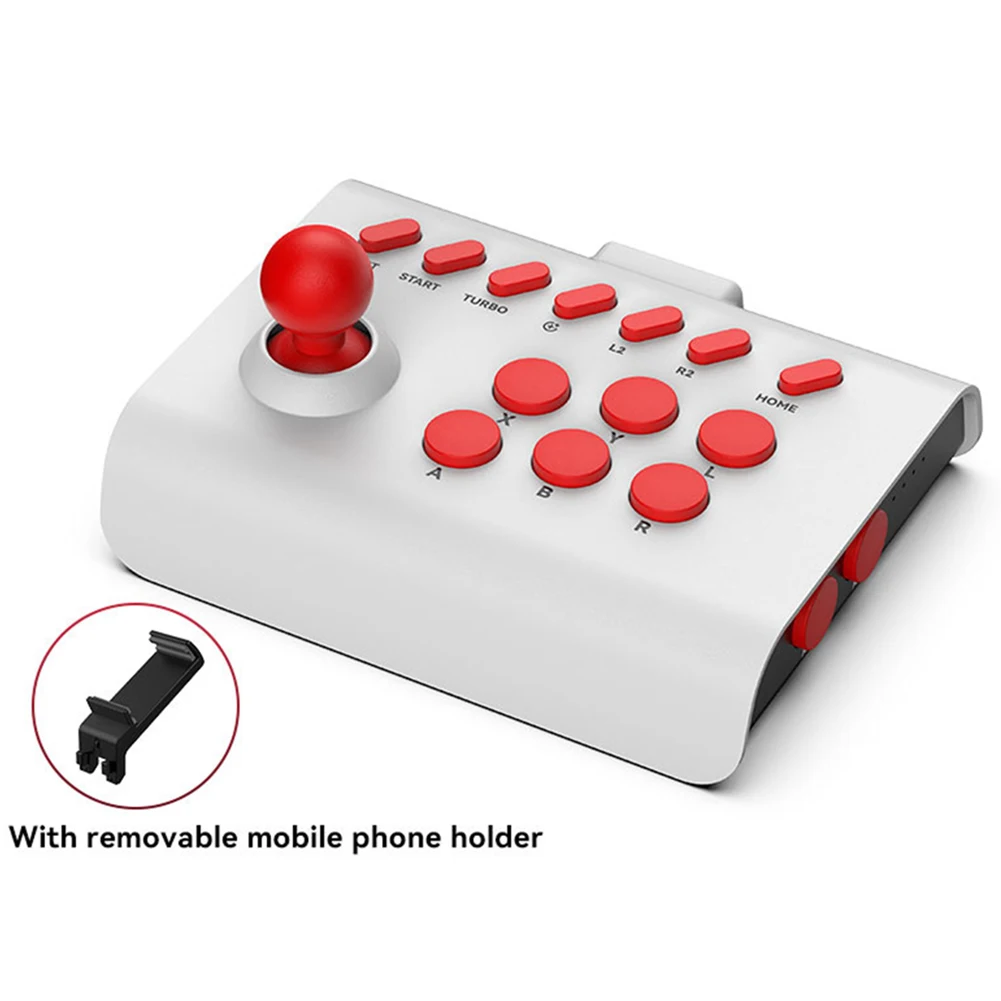This image depicts a white joystick controller equipped with various red buttons and a red joystick. The controller is designed to be versatile and portable, featuring a removable black mobile phone holder that allows the device to attach to your mobile phone. The joystick is positioned on the bottom left, adjacent to six main red circular buttons arranged in a 2x3 grid, labeled with letters X, Y, L, A, B, and R. Additionally, there are six smaller, pill-shaped red buttons angled diagonally at the top, labeled with functions such as start, turbo, L2, R2, and home. The controller also includes two extra red buttons on the side. The overall casing of the device is off-white, with its compact size comparable to a phone, enhancing its portability and ease of use.